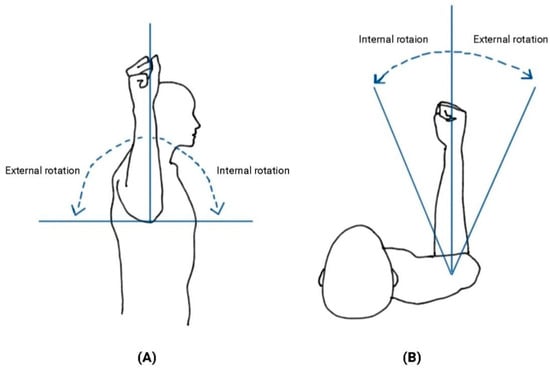The image consists of two detailed illustrations labeled "A" and "B," each demonstrating the rotational movements of the arm. 

Illustration "A" on the left shows a side view of a human figure with the arm lifted and bent at the elbow. This figure is turning to the right, with a semicircular arrow indicating the range of motion. The text "external rotation" is positioned on the left side of the semicircle, and "internal rotation" is on the right side. Both labels are in black ink, while the lines and arrows are in blue.

Illustration "B" provides a top-down view of the same figure. Here, the arm is extended straight forward. A V-shaped arrow extends from the right shoulder, with another semicircular arrow at the tips of the V illustrating the motion range. Again, "internal rotation" is marked on the left side of the semicircle, and "external rotation" on the right, with black text and blue lines.

Together, these illustrations appear to be educational or indicative of physical rehabilitation movements, depicting the external and internal rotations of the arm in different perspectives.